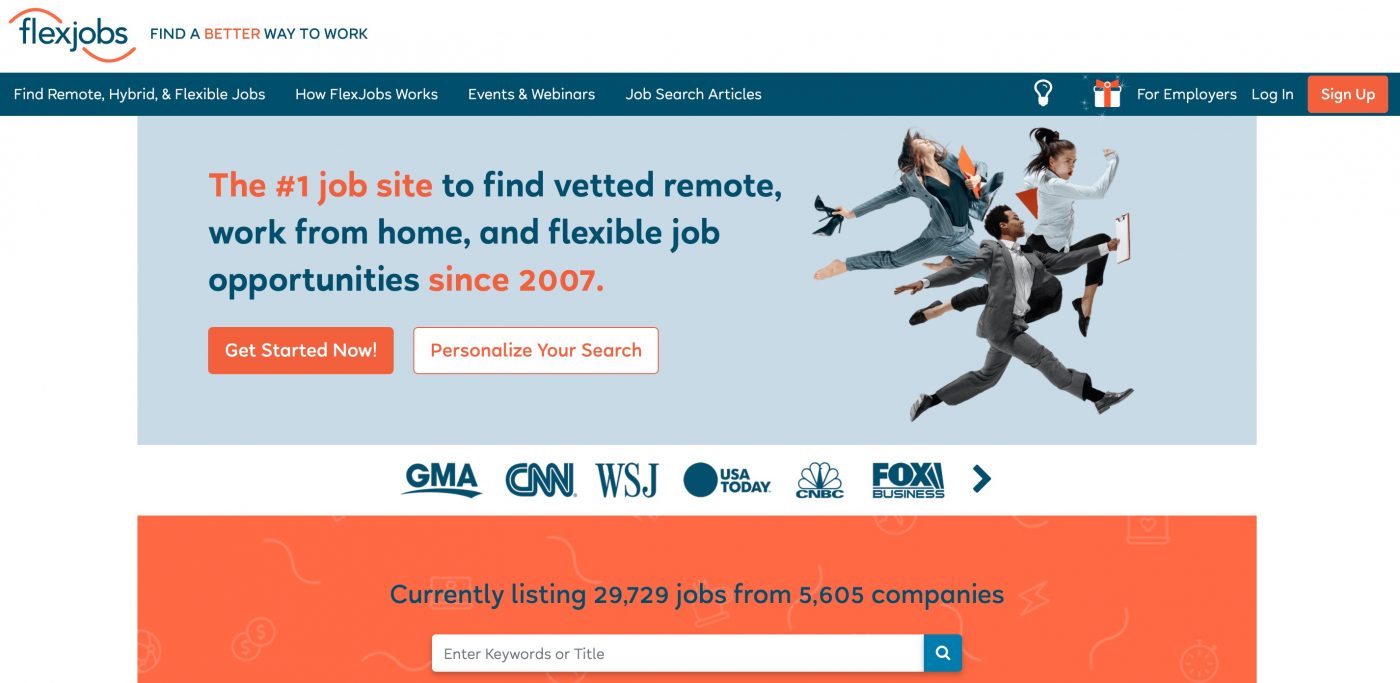The image showcases a webpage for FlexShout, featuring a detailed layout with various sections and textual content. 

At the top of the page, there is a prominent header with "FlexShout" displayed, flanked by a white background on the right, resembling a tail. This is accented by an orange line above and below the text. Beneath the header, the slogan reads, "Find a Better Way to Work," within an orange-bordered tail design.

Following this, a series of horizontal bars guide the user through different sections:

1. The first bar states, "Find Remote, Hybrid, and Flexible Jobs" in white text against an orange-tinted background.
2. The next bar is labeled, "How FlexShout Works."
3. The subsequent bar mentions, "Events and Webinars."
4. The fourth bar is dedicated to "Search Job Search Articles."

Below these bars, there's a white lightbox with a gift box image featuring a red and orange ribbon, accompanied by text for employers and a login option. Adjacent to this is an orange rectangle with white text prompting users to "Sign Up."

The page's background transitions to a light grayish-blue hue, where the main message is displayed across several lines of text:
- "The #1 Job Site"
- "Remote, Work from Home, and Flexible Job Opportunities"
- "Since 2007"

Further down, there are two prominent call-to-action boxes:
1. An orange box with white text stating, "Get Started Now!"
2. A white box with an orange border and text inviting users to "Personalize Your Search."

Below these boxes, an image of three people racing depicts the urgency of finding the right job.

At the bottom of the page, logos from notable media outlets, including GMA, CNN, WSJ, USA Today, CNBC, and Fox News, are displayed, leading into an arrow pointing to more content.

Lastly, an orange background section lists "Currently 29,729 Jobs Available for 5,605 Companies."